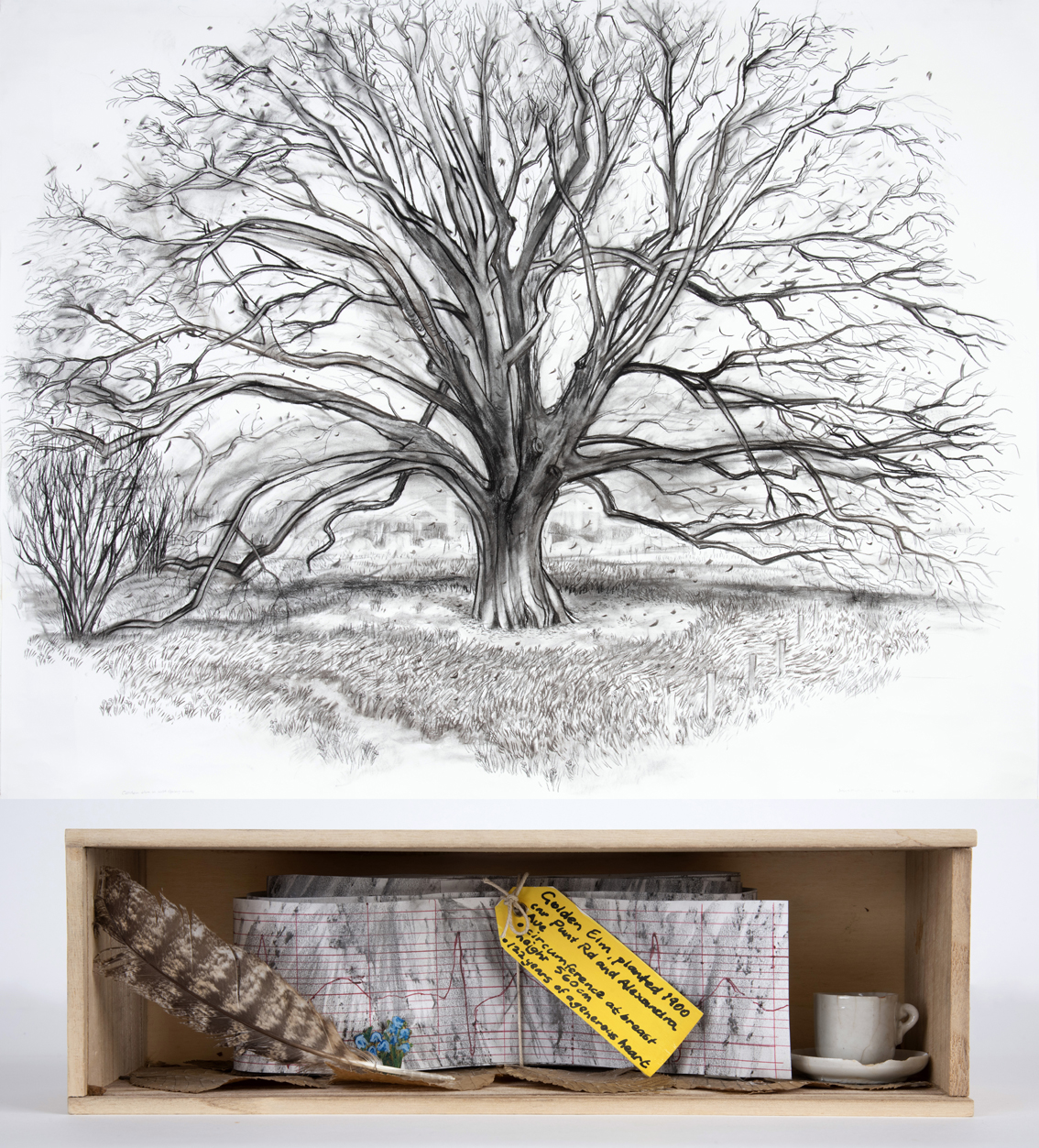The image is a composite layout in portrait orientation, divided into two distinct halves. The top half features a detailed black-and-white drawing of a very large tree, possibly a "Golden M" planted in 1900, as indicated by a yellow tag on a folded-up piece of graph paper in the bottom half. The tree, devoid of leaves, has intricate branches stretching upwards and outwards, with dashes indicating grass at its base. Below the tree drawing is a wooden cabinet with only its front open, resembling a built-in shelf. Inside the cabinet, a white cup rests on a broken white plate, next to a brown feather on the left and some blue flowers in the front. Together, these elements create a visually intriguing composition, blending botanical illustration with a still-life arrangement.